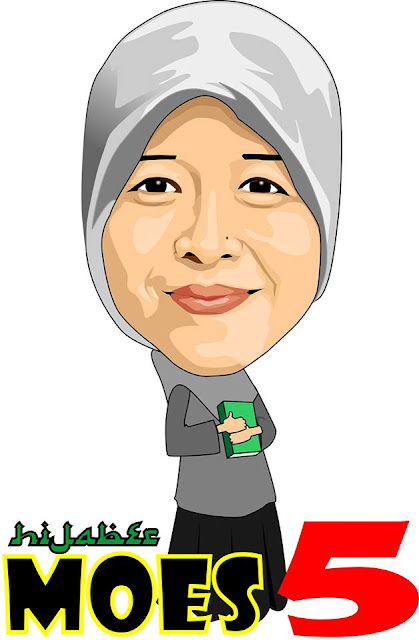This digital, cartoon-style illustration depicts a Muslim woman with light tan skin and very dark brown eyes, accentuated by thin, straight eyebrows. She is modestly smiling, and has reddish lips and a subtle nose piercing. Her exaggeratedly large head is covered in a gray headscarf with varying shades and shadows of gray, indicative of fabric folds. She wears a gray long-sleeve top paired with a black skirt. Clasped in both hands against her chest is a green book inscribed with text in a language that appears to be Arabic. Below her, additional text in black with a yellow border reads "Moes" and is juxtaposed with a large, bold red number "5".